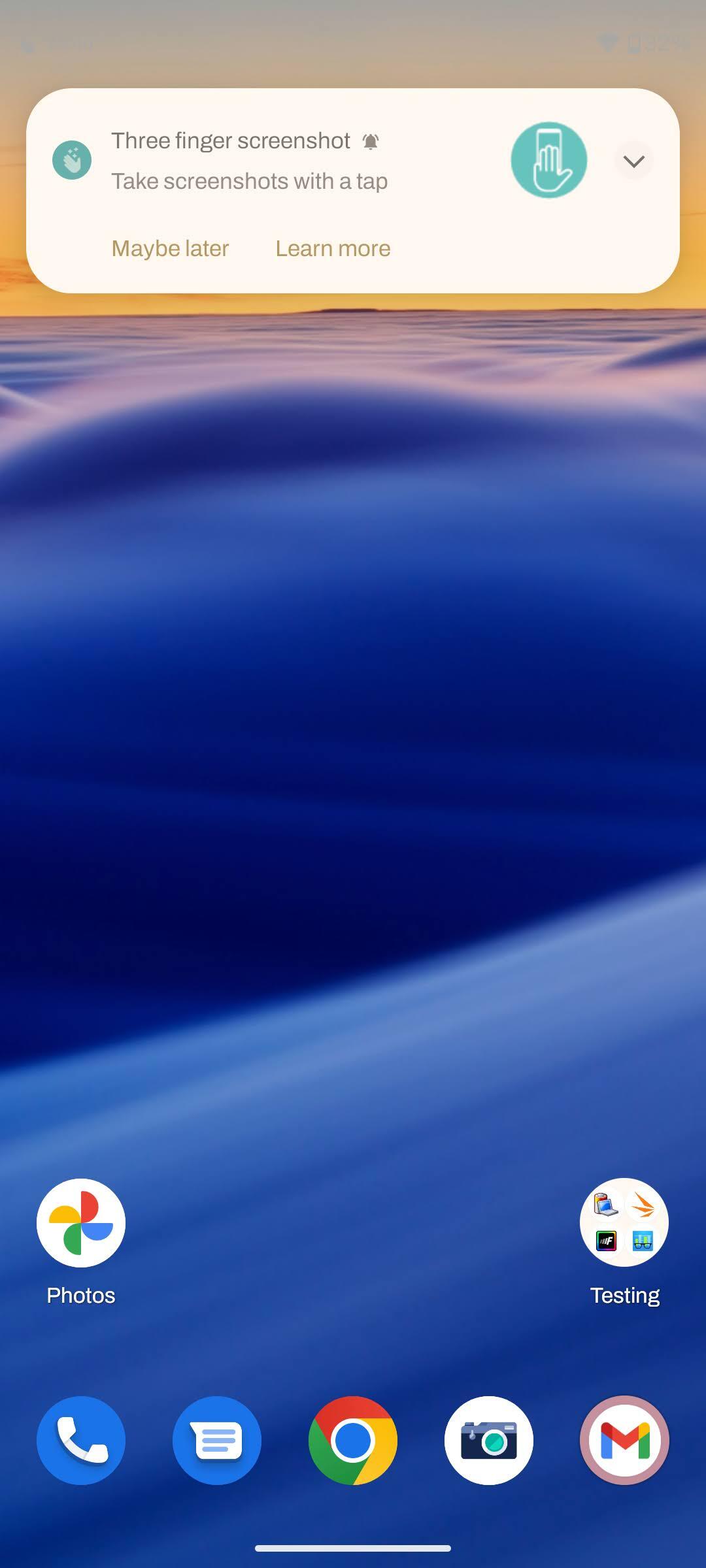The image depicts a smartphone screen featuring a background photo of fluffy white and blue clouds set against a yellowish sky gradually transitioning into light blue at the very top. Overlaying this serene background is a dialogue box at the top that reads: "Three-finger screenshot. Take screenshots with a tap." Accompanying this message is a small icon of a hand on a phone inside a green circle, with a down arrow adjacent to it. At the bottom of this dialogue, there are two clickable options: "Maybe later" and "Learn more."

The majority of the screen remains dominated by the cloud-filled background. Near the bottom, a row of icons can be seen: the first icon labeled "Photos," which appears to be the Google Photos icon, followed by a folder named "Testing" containing four smaller icons. Below this row, a dock at the very bottom houses five primary icons including Phone, Google Browser, Camera, Email, and Messaging apps. The image captures a typical smartphone interface while highlighting a new screenshot feature.